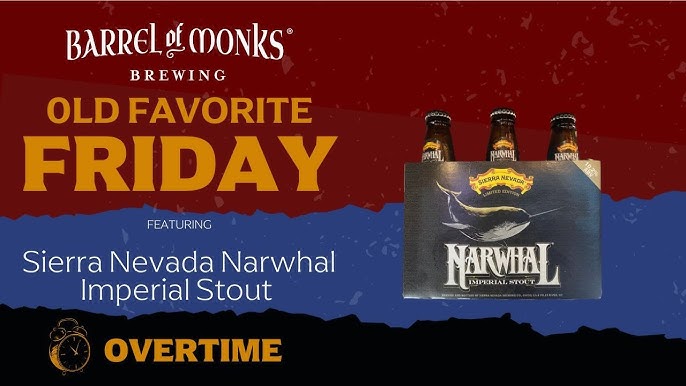The advertisement promotes Sierra Nevada Narwhal Imperial Stout as part of Barrel of Monks Brewing's "Old Favourite Friday" promotion. Divided horizontally into three color sections—maroon at the top, purple in the middle, and black at the bottom, the background features wavy, torn-like borders. On the left, white text reads "Barrel of Monks Brewing," with "Old Favourite Friday" in orange beneath it. Below this, "Featuring" is highlighted in white text followed by "Sierra Nevada Narwhal Imperial Stout." An alarm clock icon marked "Overtime" occupies the bottom left corner, encased in a yellow-orange outline. On the right side of the ad, a six-pack of the Narwhal Imperial Stout is depicted, with three visible bottles emerging from the gray pack branded with the Narwhal name in white at the bottom.